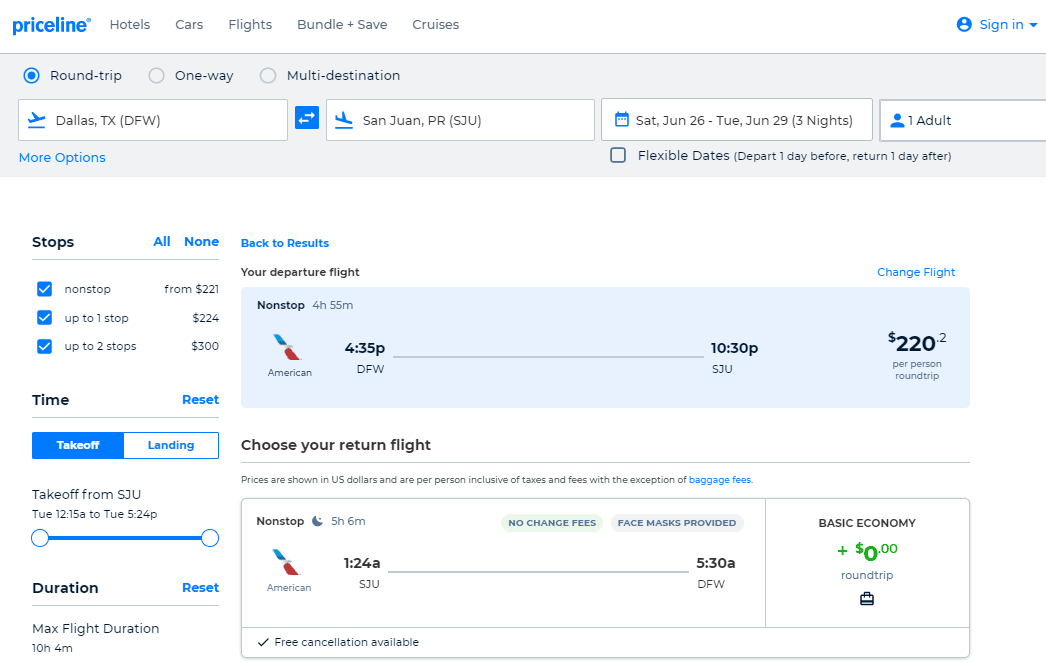The image depicts a detailed screenshot of the Priceline website interface focused on travel booking. In the top left corner, the Priceline logo is prominently displayed. Adjacent to the logo, there are five navigation categories: Hotels, Cars, Flights, Bundle and Save, and Cruises. To the far right of these categories, a sign-in option is available.

Below the navigation bar, three travel options are clearly visible: Roundtrip, One-Way, and Multi-Destination. The selected itinerary includes travel from Dallas, Texas, to San Juan, PR, with the travel dates specified from Saturday, June 26th, to Tuesday, June 29th, accounting for a three-night stay and one adult traveler.

The background transitions from light gray at the top to white below. On the left, there is a section labeled "Stops" with three selectable options, all of which are currently selected, along with the corresponding prices displayed to the right. Below this section is the "Time" filter accompanied by options to reset, set takeoff, and landing times.

In the bottom left corner, the "Duration" filter is set with a maximum flight duration of 10 hours and 4 minutes. Centralized on the page, the option to navigate back to results is highlighted in blue. The departure flight details are shown on a light blue background, indicating a flight time from 4:35 PM to 10:30 PM, with a cost of $220 per person. The return flight details are displayed below, showing a flight time from 1:20 AM to 5:30 AM. The return flight's fare class is noted as Economy with $0 in green text, all encased within a rectangular gray outline.